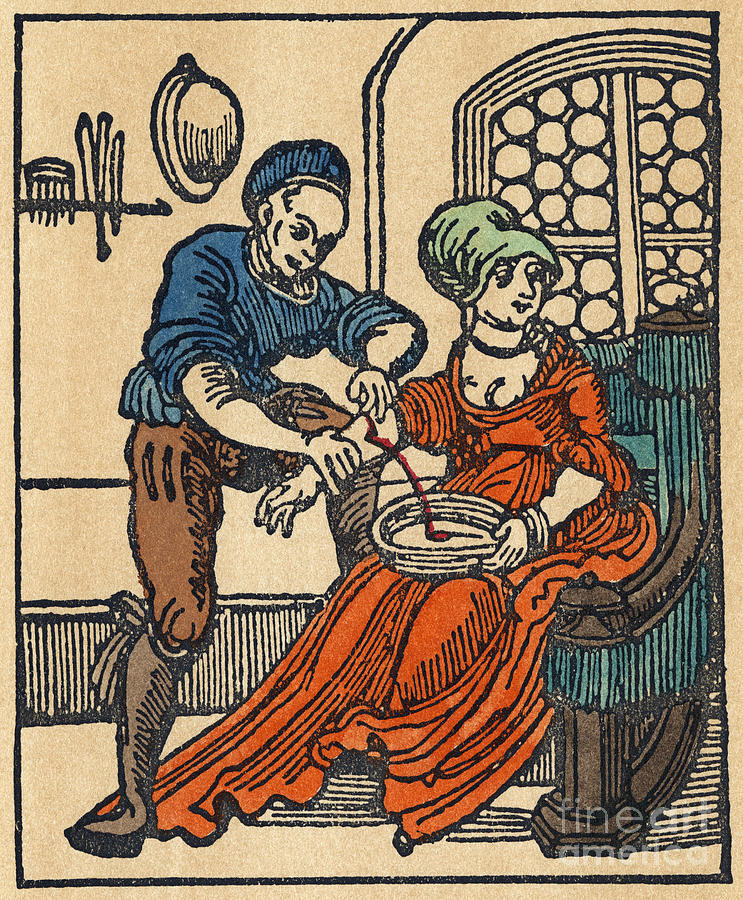The image is an intricately detailed drawing reminiscent of the medieval or renaissance period, possibly from the 1800s. It features a man and a woman positioned against a beige background adorned with a shelf and a hat hanging above it. The man, possibly a doctor or apothecary, is dressed in a blue shirt with half-length sleeves, brown pants, brown boots, and a blue cap. He stands over a woman seated in a large, ornate green chair, with his left leg propped on the chair. The woman is elegantly clad in a voluminous red gown that extends to her ankles, and her hair is styled in an upswept bun or a green turban. She holds a wide bowl in her lap into which blood flows from her right forearm. Her right arm, bare from the elbow down, is held by the man as the blood is drawn. The composition of the scene, including the awkwardly depicted bosom and voluminous fabric of her gown, gives it an old-timey, engraved quality. In the far corner of the image, the words "Fine Art America" are inscribed.